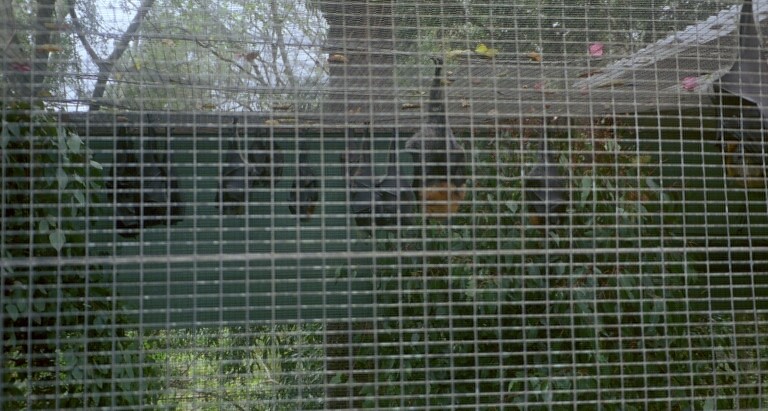The photograph features a detailed outdoor zoo exhibit with a tightly-knit light gray metal cage enclosing the space. The cage has small rectangular openings, including across the ceiling, ensuring the creatures inside cannot escape, while still allowing visibility and natural daylight to flood in. Inside, the area is teeming with lush green plants and leafy vegetation, providing a rich, natural backdrop. Clearly visible are black bats hanging from the top of the cage, one of which is particularly notable for the orange coloring near its head. Tall trees grow in the background, further enhancing the natural ambiance of the exhibit. The intricate cage structure ensures the safety and containment of the enclosed animals while allowing visitors a clear view of the interior.